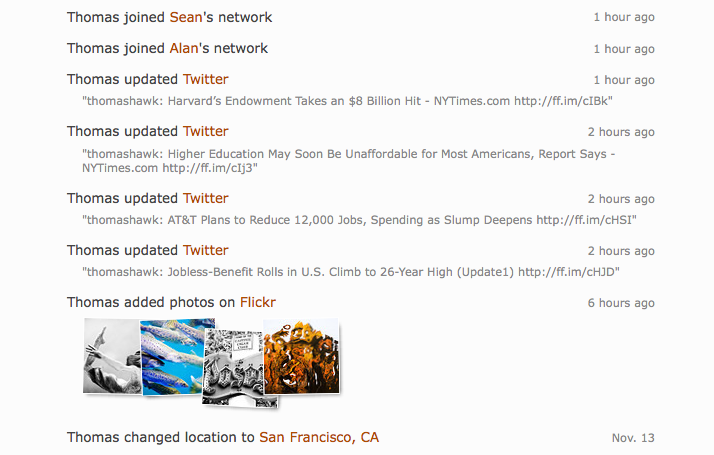The image presents a detailed timeline of Thomas John Allen's recent online activities, divided into two columns. In the top row of the left column, it starts with "Thomas John Allen's lab work, one hour ago." Sequentially, it continues with "Thomas joined Sean's network one hour ago," "Thomas joined Alan's network one hour ago," and "Thomas updated Twitter one hour ago" with a story from the New York Times about Harvard's endowment taking an eight billion dollar hit. Further down, it notes that Thomas updated Twitter two hours ago with another higher education story, followed by another post about AT&T planning to reduce 12,000 jobs due to a slump. Continuing in the same timeframe, another update highlights that jobless benefits rolls in the US have climbed to a 26-year high. Six hours ago, Thomas added photos on Flickr, featuring four small images—the first being black and white and the second blue with some white fish. The timeline also notes that Thomas changed his location to San Francisco, California on November 13th. This thorough record encapsulates Thomas’s recent social media updates and engagements across different platforms.